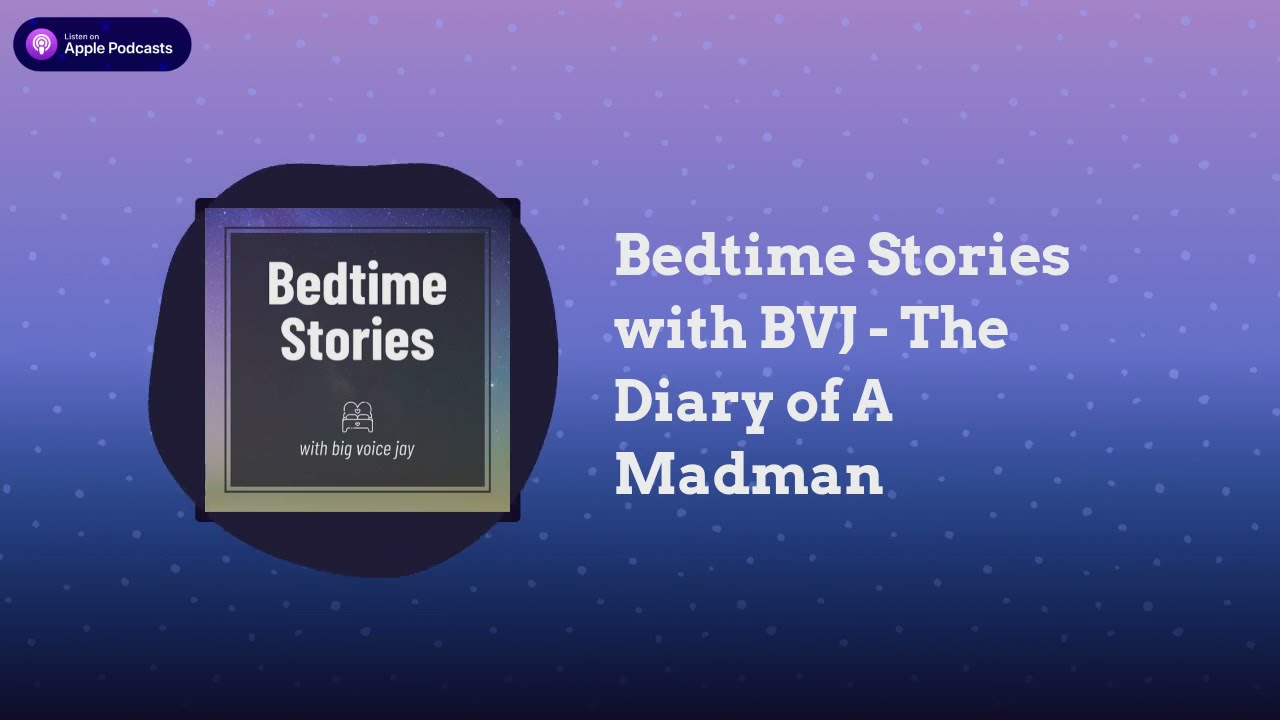The image features a visually appealing, digitally created advertisement or banner ad for a podcast. The background starts with a rich purple hue at the top, gradually transitioning through shades of blue to a deep navy at the bottom, evoking the look of a nighttime sky sprinkled with small star-like dots. 

In the top left corner, a small oblong shape contains the purple Apple Podcasts icon beside the text "Listen on Apple Podcasts". Dominating the center of the image is an album cover-like graphic. This graphic includes a dark box outlined with purple and green hues, displaying the text "Bedtime Stories with Big Voice Joy". To the right of this central box, the white text "Bedtime Stories with BVJ: The Diary of a Madman" stands out against the background.

The composition and color scheme include shades of black, white, purple, blue, and traces of green, creating a cohesive, attractive advertisement specifically tailored to promote the podcast effectively.